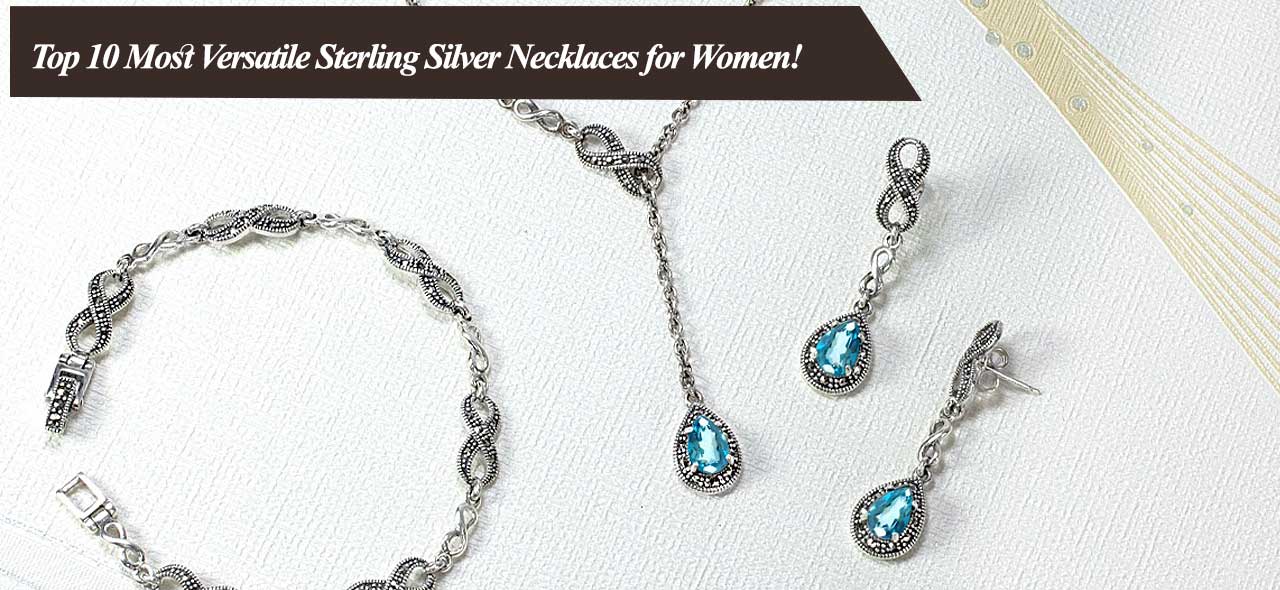This image appears to be from a magazine article on jewelry, showcasing a matching set of sterling silver pieces for sale. The set includes a drop necklace, a pair of pierced earrings, and a bracelet. The necklace and earrings feature teardrop-shaped blue stones, possibly blue topaz or light blue turquoise, set in silver. The bracelet, devoid of any stones, includes a number 8 design adorned with small diamonds or rhinestones. The pieces are elegantly arranged on a soft, white cloth or paper towel background. In the upper left corner, a black ribbon with white lettering reads, "Top 10 most versatile sterling silver necklaces for women." There is no price or website provided for purchasing these items.